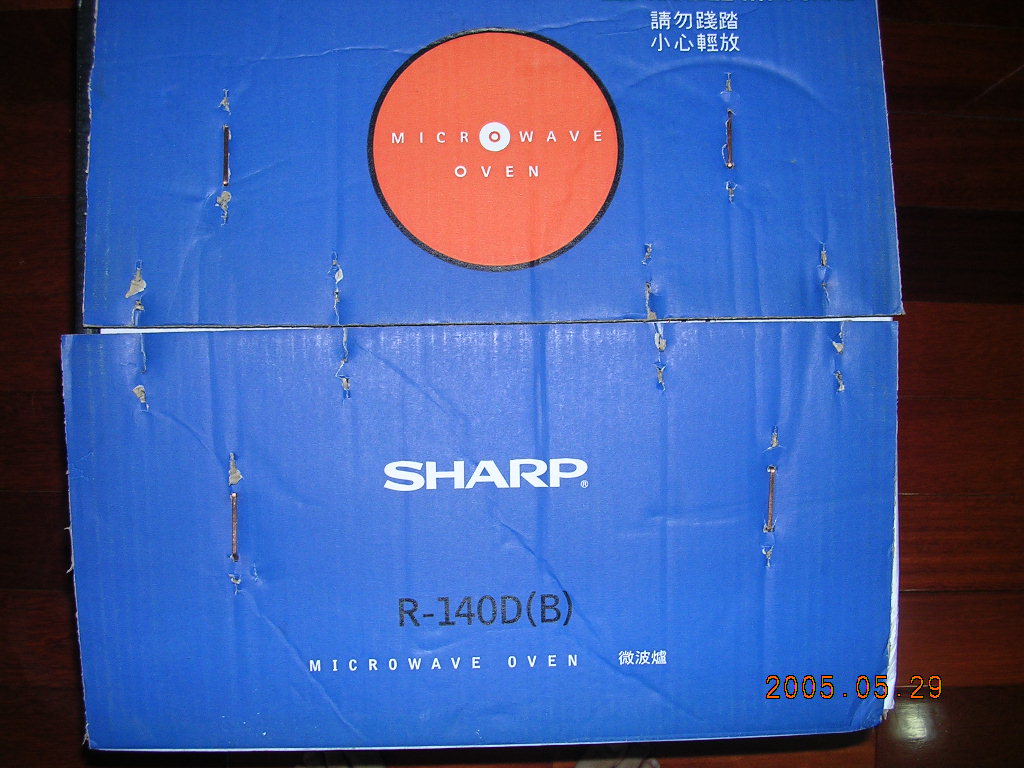This overhead, color photograph captures the close-up of a blue microwave oven box taken with an old-style film camera, as evidenced by the orange analog date stamp in the bottom right corner reading "2005.05.29." The top flap of the box prominently features a large red circle, bordered in black, enclosing the words "microwave oven" in white font. Adjacent to this circle, in the top right, are two rows of Chinese or Japanese characters. The sturdy box is secured by several copper-colored staples, some of which have left noticeable marks where they were removed. On the bottom flap, the brand name "SHARP" is displayed in large white letters, along with the model number "R-140D" followed by "(B)" in black font, and the repeated designation "microwave oven" in smaller white text, accompanied by more Chinese or Japanese characters. The ambient light from above casts a reflection on the box's surface, suggesting it might be placed on a tabletop.